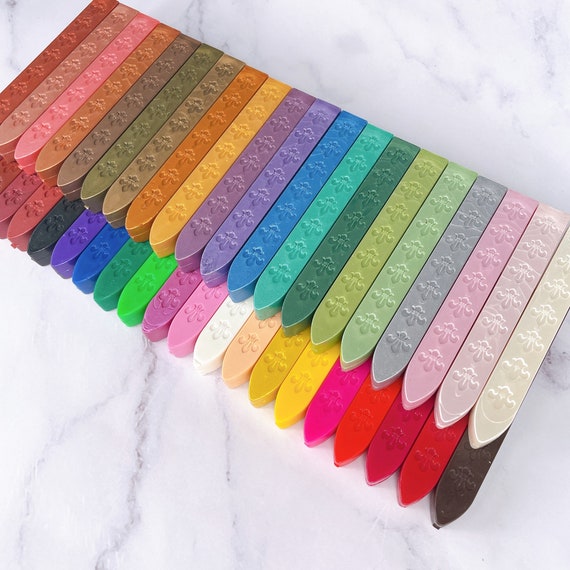The image depicts a collection of long, thin items, possibly crayons or markers, arranged in two layers on a light pink or purple marble surface. These items are rectangular with pointed ends and are presented in a wide array of colors. The top layer features an assortment of whites, greens, blues, yellows, and oranges, while the bottom layer includes deeper shades such as dark brown, dark red or burgundy, bright green, and bright blue, along with a variety of other hues including red, pink, ivory, tan, sage green, aqua blue, violet purple, and light gray. Some of the objects have fleur-de-lis designs on them. The photo is taken from an overhead perspective, emphasizing the vibrant color diversity and intricate arrangement on the marble background.